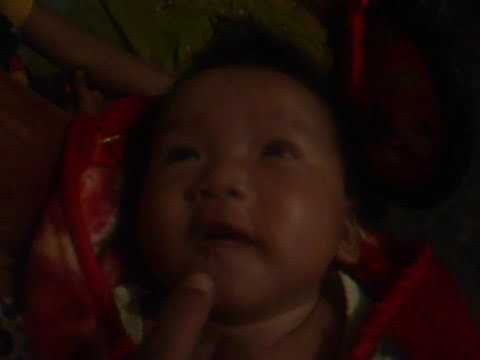This blurry, close-up photograph captures the curious gaze of an Asian infant, likely just a few months old. Centered in the image, the baby’s round face, with chubby cheeks and wide-open, dark eyes, looks slightly upward and toward the top left. The child's mouth is partially open and the child's wispy, fluffy dark hair contrasts with its caramel-colored skin. A prominent adult finger gently touches the baby’s chin, suggesting interaction, perhaps with a parent. The infant is wrapped in a fuzzy red blanket adorned with black and white patterns, providing a cozy frame on both the left and right sides of the baby's head. The child appears to be dressed in a white onesie beneath the blanket. The background is very dark, perhaps indicating the photo was taken indoors, possibly at night, in what might be the baby's room. The overall reddish-orange hue of the image, combined with its low resolution, gives it a soft, almost dreamlike quality.